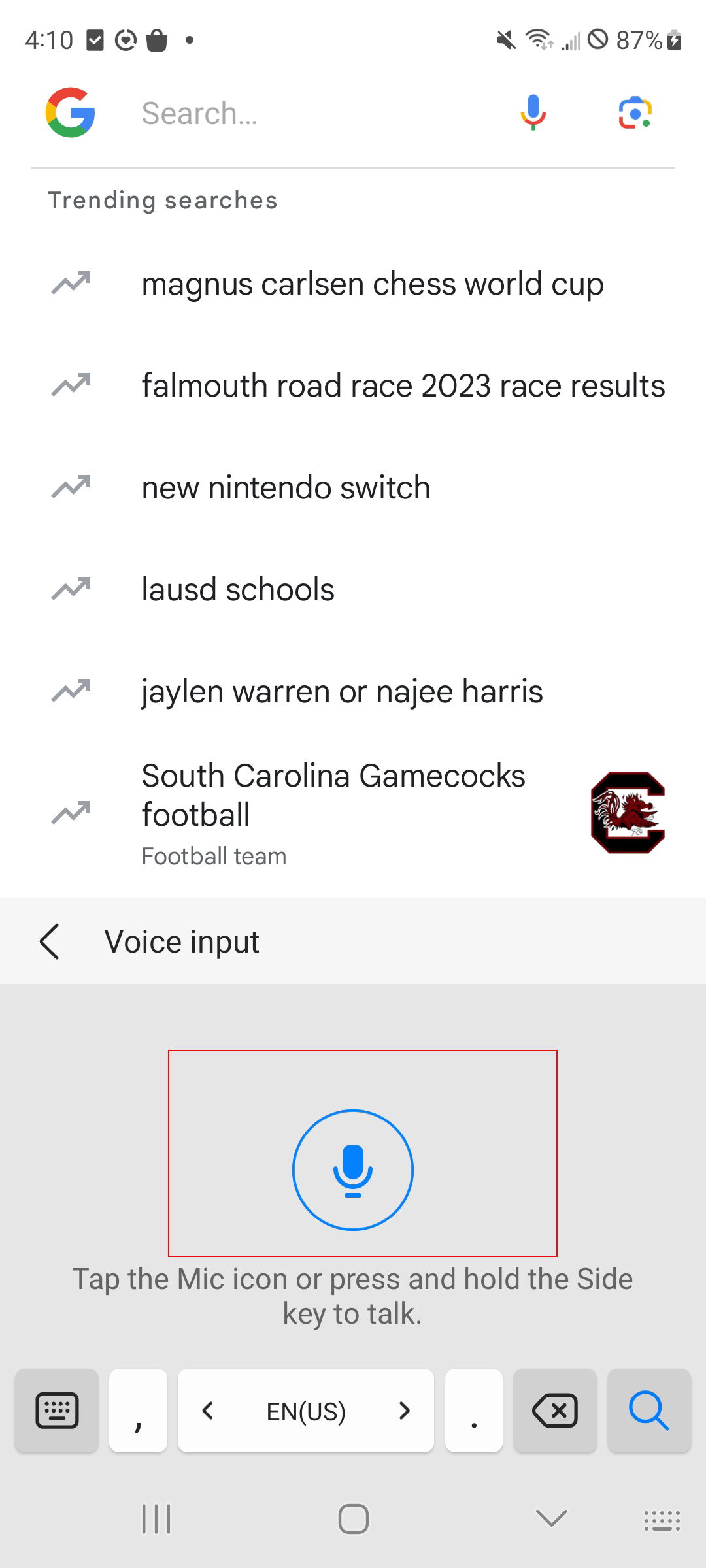Sure, here is a cleaned-up and detailed caption:

---

This image is a screenshot of a Google search page, likely from the Google search app. At the top of the screen, it is noted that the time is 4:10 PM, the device is on Wi-Fi with a relatively weak cellular connection, the volume is muted, and the battery level is at 87%. The familiar icons for microphone and camera for voice and image searches are prominently displayed. 

Underneath a fine gray divider line, the section labeled "Trending Searches" appears, denoted by a small upward-pointing arrow, and includes a list of popular searches. The top search is "Magnus Carlsen Chess World Cup," followed by "Fall Mouth Road Race 2023 Race Results," "New Nintendo Switch," "LAUSD Schools," "Jalen Warren or Najee Harris," and "South Carolina Gamecocks Football."

Additionally, the user has engaged the voice search functionality, indicated by the microphone icon within a dimmed gray box that instructs, "Tap the mic icon and press and hold the side key to talk." This feature can either assist in verbal queries or potentially record ambient sounds for Google to interpret and provide relevant search results.

---

This description covers all major aspects of the screenshot, providing a thorough and coherent understanding of the content and context.